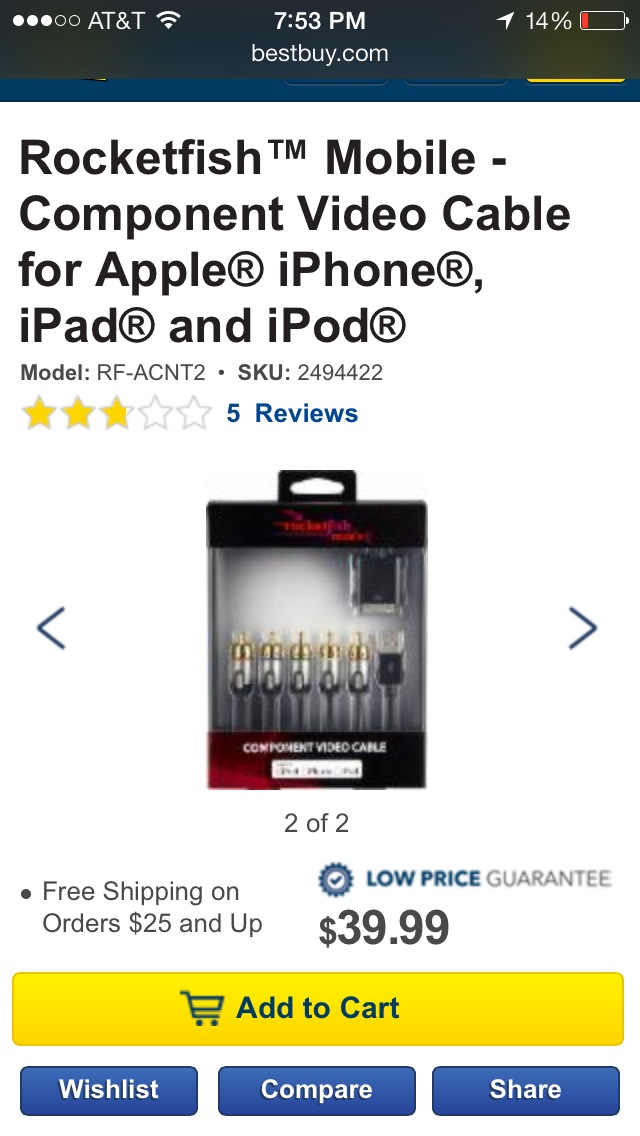This is a screenshot from an iPhone showcasing an item for sale on bestbuy.com. At the top, a black bar displays "AT&T," the time (7:53 PM), and the battery percentage at 14%. Below that, on a white background, is a description in large black letters: "Rocketfish Mobile Component Video Cable for Apple iPhone, iPad, and iPod." The model number is RF-ACNT2, and the SKU is 2494422. The product has received an average rating of nearly three stars out of five based on five reviews.

A central image features the packaged product, showing six cables within a predominantly gray box with a black horizontal stripe at the top. Further down, a yellow banner prominently states "Add to Cart" in blue letters. Below this yellow bar are three blue buttons labeled "Wishlist," "Compare," and "Share." Additional details include a note about free shipping on orders over $25 and a low price guarantee, indicating the item is priced at $39.99.